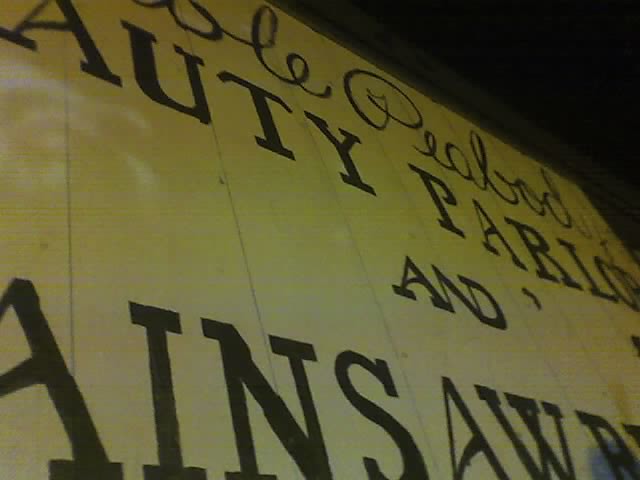The image depicts an older, unlit billboard-style sign set against a night sky, making the surroundings appear black. The billboard has a yellowish background with text in black or brown. The top portion of the sign features cursive text that appears to spell "Peabody," though the text is somewhat hard to read. Beneath it, there are blocky, black capital letters partially obscured, potentially reading "Autie Parlor" and possibly "Ainsaw." The sign seems to be mounted on vertical wooden planks, reinforcing its classic and weathered appearance.